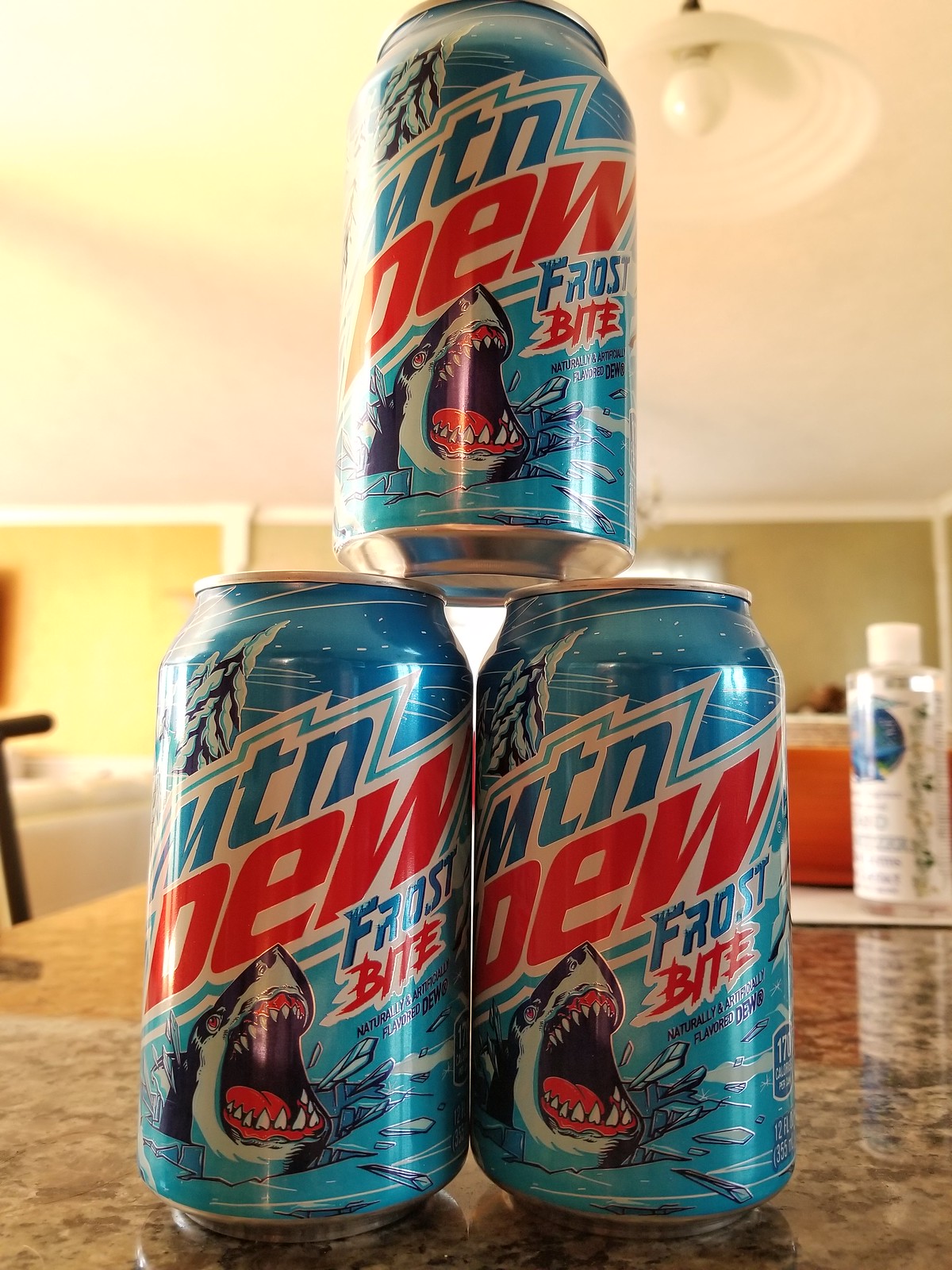This photograph, taken from a low angle close to the top of a countertop, captures a section of what appears to be a kitchen. The countertop, which looks to be made of marble or granite in a brown, creamy hue, features a small pyramid arrangement of three light blue Mountain Dew Frostbite cans stacked with two at the bottom and one on top. The cans are positioned with their logos facing forward, displaying the words "MTN DEW" in blue and red, respectively, and "Frost Bite" below, with "Frost" in blue and "Bite" in red. The design includes an image of a shark breaking through ice, its open mouth revealing red gums, a red tongue, and white teeth. In the background, against a white wall, a yellow-painted cabinet can be seen, along with a round white light fixture hanging from the ceiling in the upper right corner. Additionally, there is a clear plastic bottle next to a red object on the back right side of the countertop.